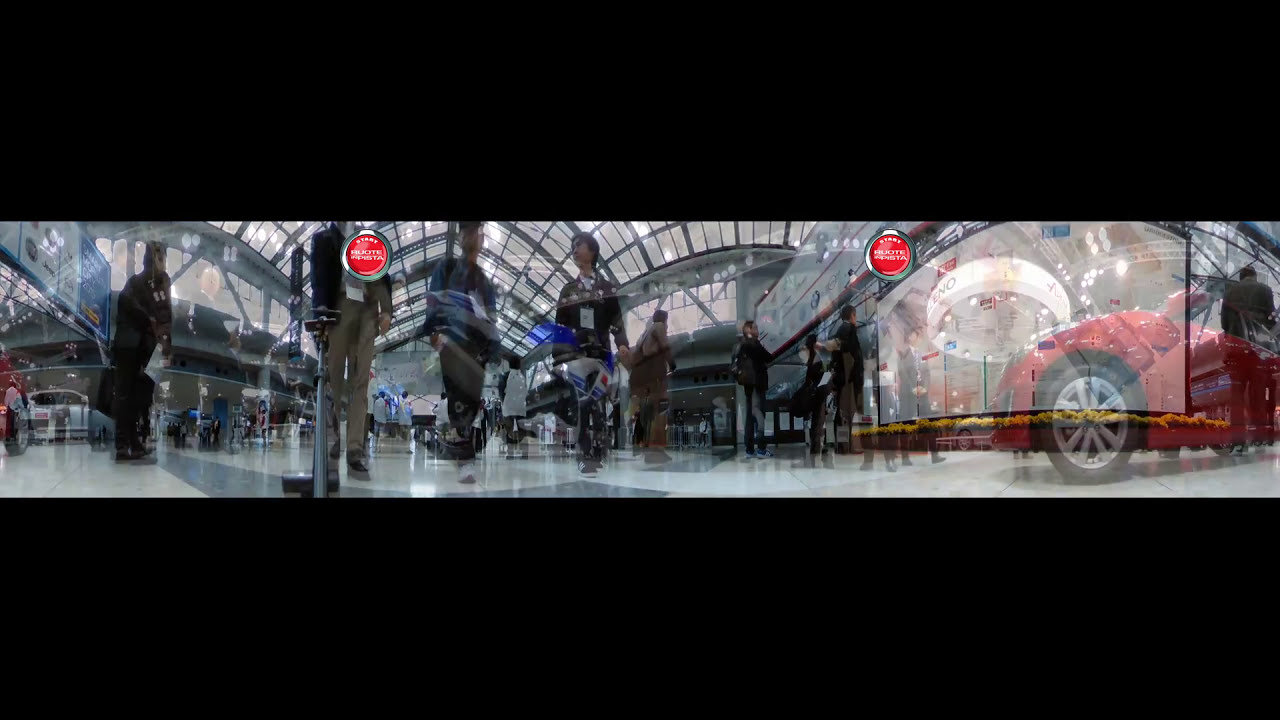This wide panoramic photograph captures the bustling ambience of a terminal, possibly an airport or train station, distinguished by its expansive glass atrium ceiling that bathes the scene in natural light. The flooring, arranged in a distinctive pattern of white and black tiles, reflects the movement of numerous people, some adorned with badges around their necks, navigating the busy space. Despite the slightly blurry and abstract rendering, several features are distinct: a red car appears to the right, possibly mirrored by the glass surfaces, while a distant silver truck is discernible on the left. Red signs hang overhead, though their inscriptions remain illegible, adding to the layered, somewhat surreal quality of the image. In the center, a figure on a bicycle and several male figures are vaguely visible, contributing to the dynamic and multifaceted nature of the scene.